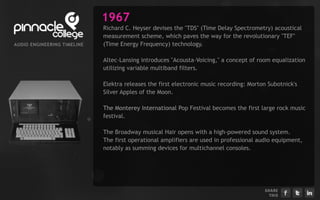This image appears to be an informational slide about a vintage computer from 1967, created by Pinnacle College. The slide is part of a website commemorating the history of audio engineering developments from that year. The computer is depicted on the left-hand side of the slide: a large, boxy unit with a light gray metal frame and a small CRT television screen on the left. The black front panel contains a docking area for a keyboard, which is light gray with black framing and keys. Above the computer, Pinnacle College's white logo is visible. On the right-hand side, a black box contains multiple paragraphs in light gray text that are too small to read clearly, except for the pink-colored year 1967. Some content mentions groundbreaking technologies of the era, including Richard C. Heiser's TDS time-delay spectrometry scheme and the first electronic music recording by Morton Subotnick. At the bottom right of the slide, social media links to Facebook, Twitter, and LinkedIn are also visible.